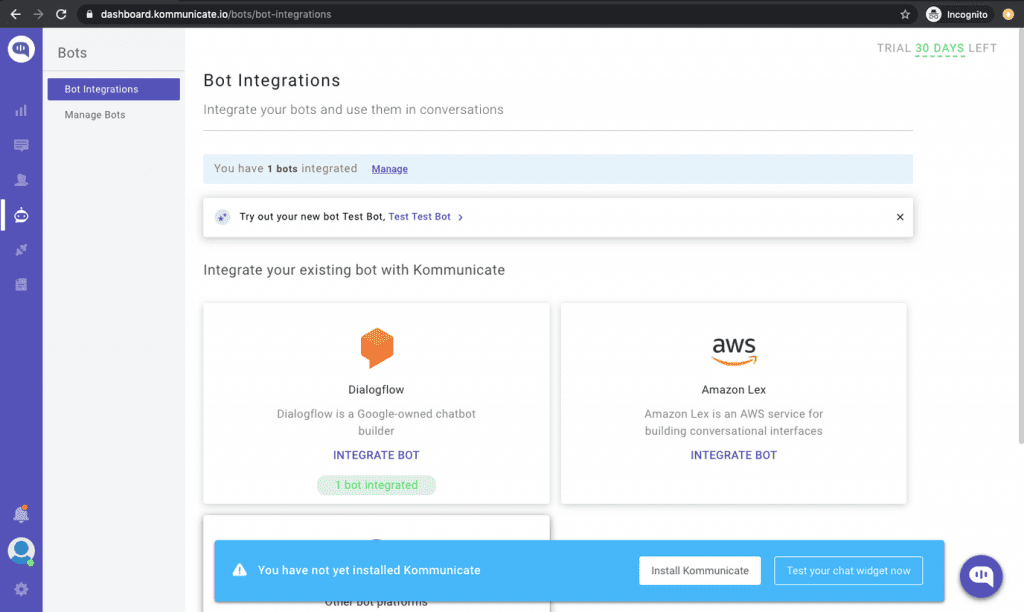The image displays a web browser interface within an incognito window. At the top, a black border houses several navigation icons including back, forward, and refresh buttons, alongside an unreadable URL. 

On the top right corner, the incognito mode icon is visible. Below this, on the left side, there's a vertical purple sidebar running from the top to the bottom of the page. This sidebar features multiple icons, such as signal indicators, a notification bell, and a generic profile picture.

Adjacent to the purple sidebar, there's a gray box labeled "box." Directly beneath it, a rectangular dark blue section contains some unreadable text, followed by additional smaller text that is also illegible due to blurriness. To the lower right area, there is a section titled "Bot Integrations," with a description that reads, "Integrate your bots and use them in conversations." A cut-off section follows below this text.